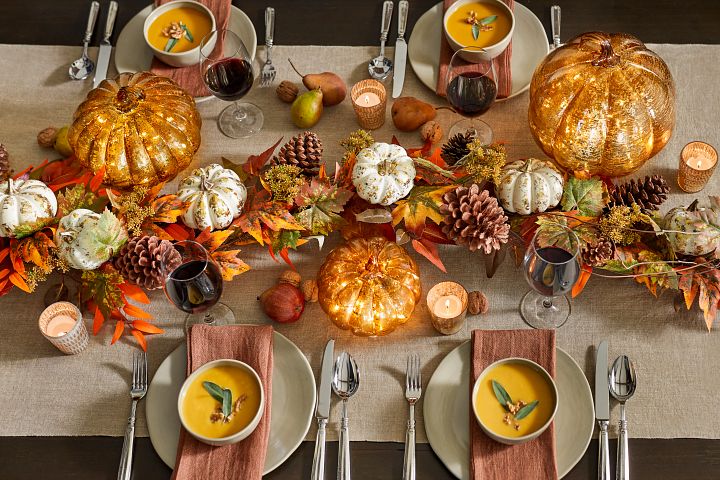The table is set for an autumnal meal, adorned with an array of festive fall decorations that create a warm and inviting atmosphere. A tan tablecloth hosts four identical place settings, each comprising a white plate with a pale red napkin folded neatly in the center, topped by a white bowl filled with an acorn-colored soup, likely pumpkin soup. The soup is garnished with green herbs and small bay leaves. Each place setting includes a shiny silver fork on the left, and a knife and spoon on the right. 

Amongst the place settings are four glasses of red wine, one per plate, and a candle next to each setting, casting a cozy glow. The centerpiece of the table features a collection of autumn-themed decorations including various-sized pumpkins—some are white and others are amber-colored, illuminated either from within or by reflecting ambient light, giving them an enchanting glow. Scattered around these pumpkins are autumn leaves, pine cones, acorns, walnuts, and a pear, enhancing the seasonal charm. The entire setup is beautifully complemented by the natural elements and the warm hues of the decorations, creating a picturesque scene perfect for a harvest feast.